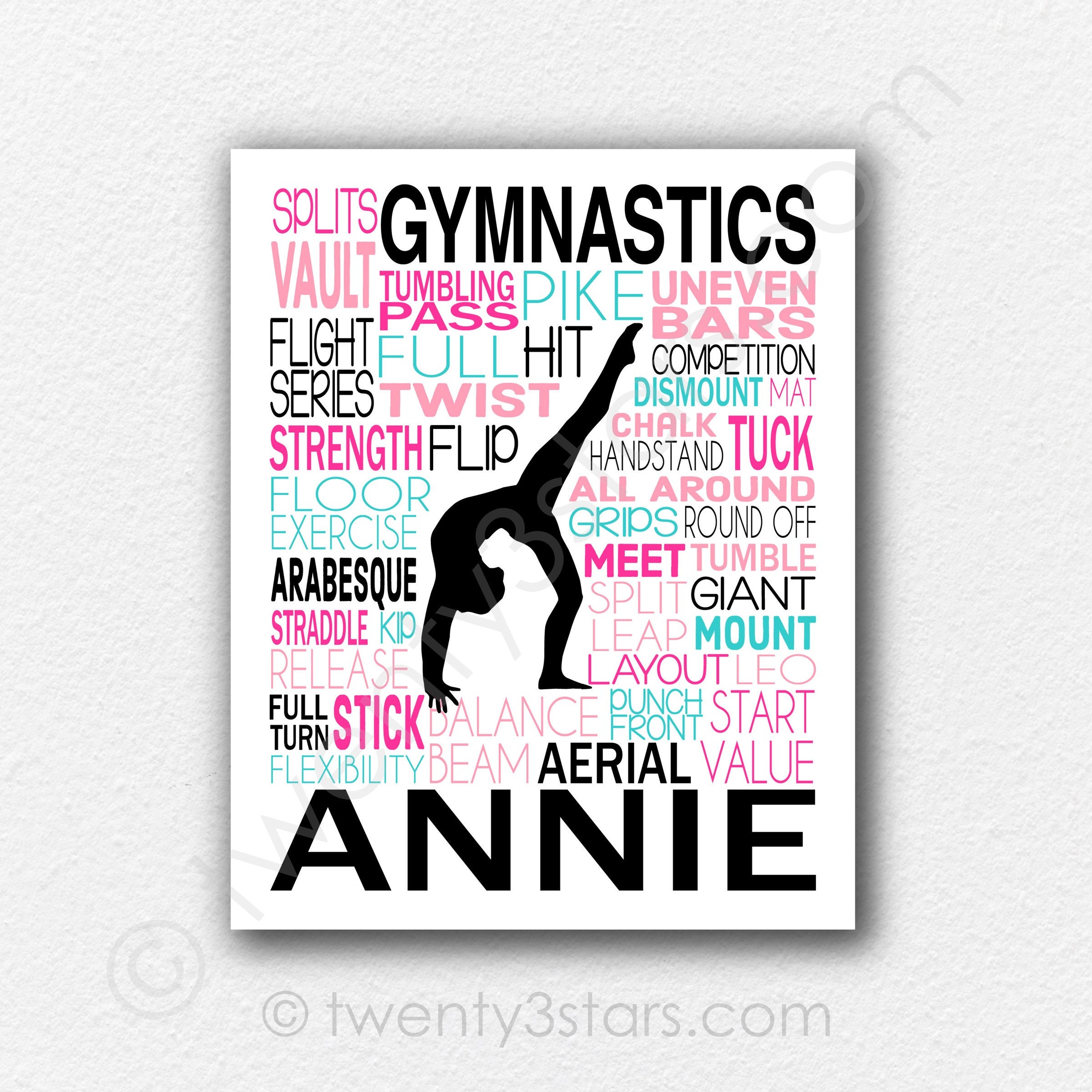The image is an advertisement for a gymnastics class featuring a white, square poster set against a light lavender background. At the very top of the poster, in bold black all-caps, is the word "GYMNASTICS." Below this, in the center, is the silhouette of a woman performing a gymnastic pose, with one leg extended straight into the air, while the other remains on the ground and her hands touch the floor. Surrounding the silhouette are various words in pink, blue, and black, listing gymnastics-related activities and skills such as "splits," "vault," "tumbling," "pike," "uneven bars," "strength," "flip," "dismount," "giant," "meet," and many more. Prominently displayed in large, bold black letters towards the bottom of the poster is the name "ANNIE." At the very bottom of the poster, a trademark symbol is present along with the website address "23stars.com," where "20" is spelled out and "3" is numerical.